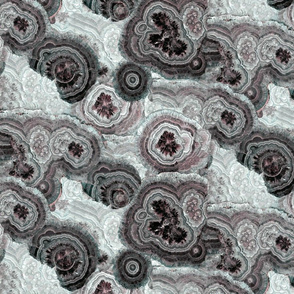The photograph captures a detailed cross-section of a geode, showcasing a mesmerizing pattern of concentric circles and nodular shapes. Predominantly set against a white matrix, the image reveals clusters of geodes in varying colors such as dark gray to black, pink, purple, and a deep burgundy hue. The intricate layers and swirls resemble artistic renderings of clouds, adding an additional layer of visual complexity. Some elements of the composition may remind viewers of germ or bacteria clusters, but the primary focus remains on the dazzling array of geode formations with their rich, midnight and purple-toned interiors.